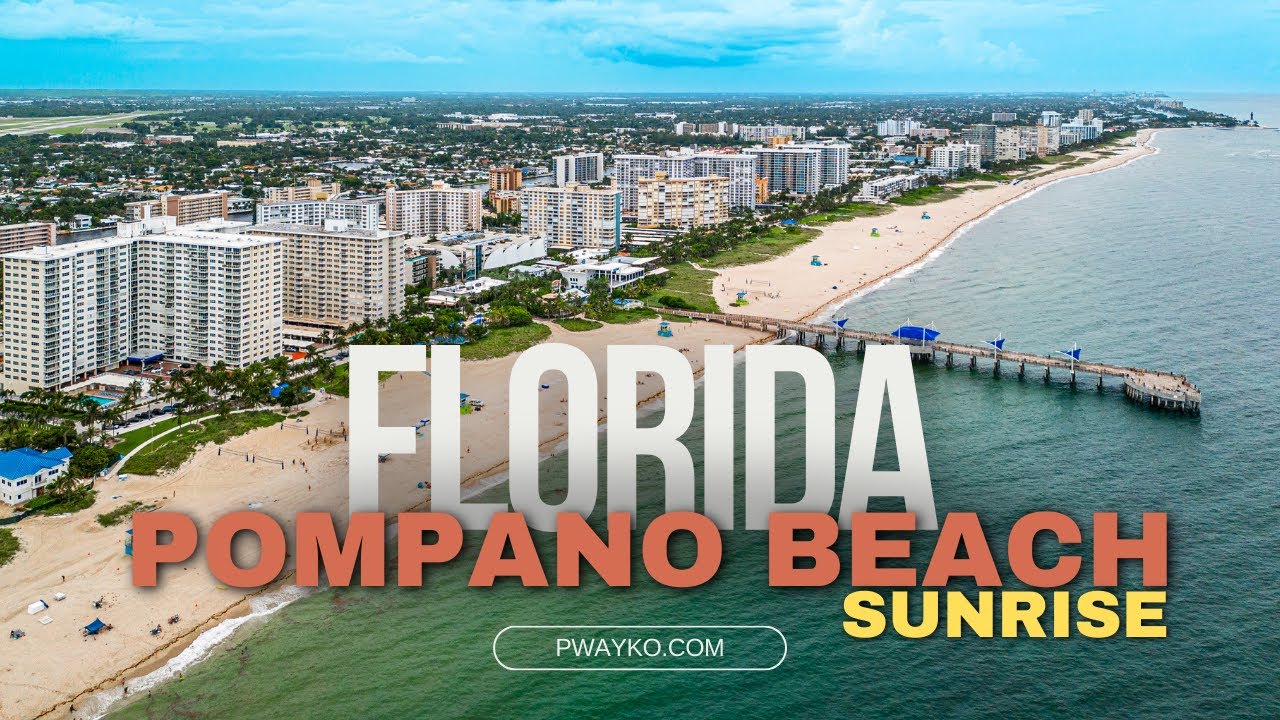The image appears to be an advertisement or postcard depicting a scenic aerial view of Pompano Beach, Florida, at sunrise. The sky is a brilliant blue adorned with white clouds. The coastline features a pristine, sandy beach bustling with a few people under blue canopies and umbrellas. A prominent wooden pier with blue flags extends into the ocean, where a couple of blue boats with white tops are docked. Large, skyrise buildings, likely hotels, populate the shoreline, surrounded by lush green areas and further complemented by distant houses and trees. In the center, the text reads "Florida" in white, "Pompano Beach" in red, and "Sunrise" in yellow, enhancing the inviting ambiance of the scene. At the bottom center, an elongated white oval hosts the web address "pwayko.com" in white font, adding to the promotional feel of the image.